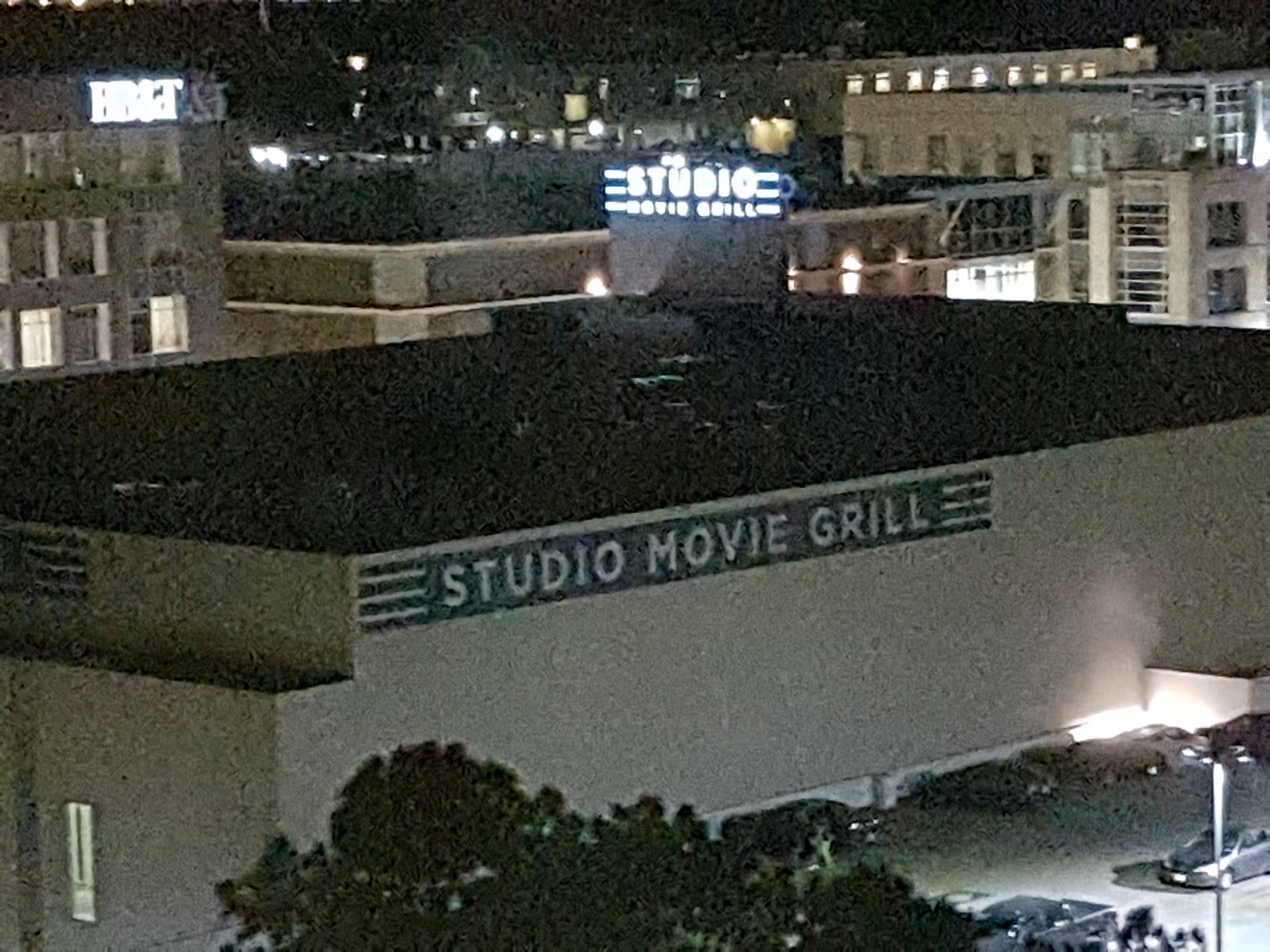A grainy photograph captures the exterior of a large building identified as the Studio Movie Grill. The building’s name is prominently displayed at the top in dark paint with bold white letters. Additionally, a neon sign on the side reads "STUDIO" in large, luminescent letters, followed by "Movie Grill" underneath. Surrounding the cinema is a parking lot, with parked cars visible, and an urban backdrop of industrial-style buildings. An office building with an illuminated sign is also in the frame, although the sign’s text is obscured due to the brightness and angle of the shot.